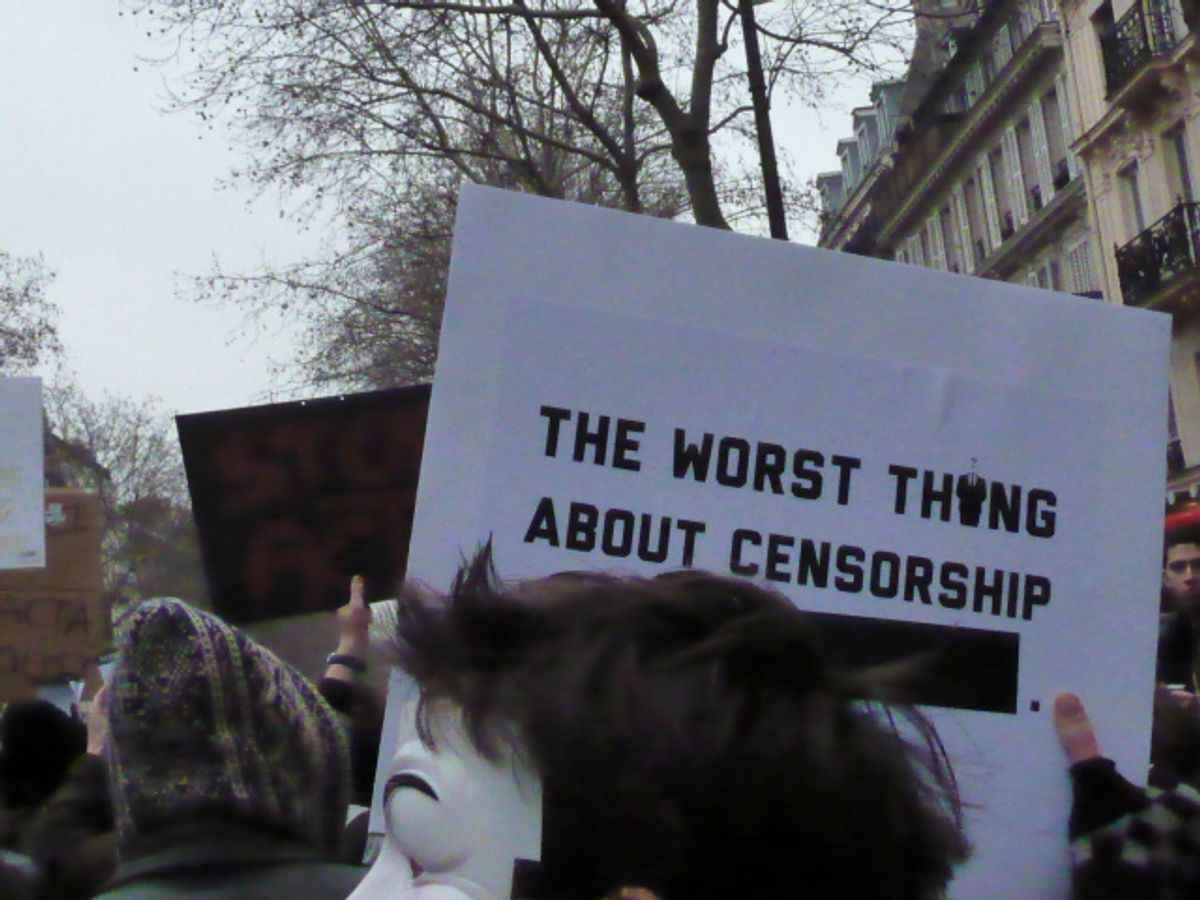This detailed photograph captures a vibrant daytime protest taking place in an urban setting, characterized by old stone brownstone buildings and leafless trees against a clear sky. The crowd is predominantly facing away from the camera, with one prominent figure in the forefront—a person with long brown hair, who is holding a white sign that reads, "The Worst Thing About Censorship," with an incomplete line of text beneath. Additionally, a masked individual, likely associated with the Anonymous group and wearing a white mask with black eyebrows, stands out close by. The crowd displays a diverse array of signs, varying in color and material—some are red and black, others are plain cardboard, and some are black and white. Another participant, with their head covered, holds a black sign that partially reads "STO" in red letters. The image is densely packed with demonstrators, each contributing to the dynamic and impassioned atmosphere of the protest.